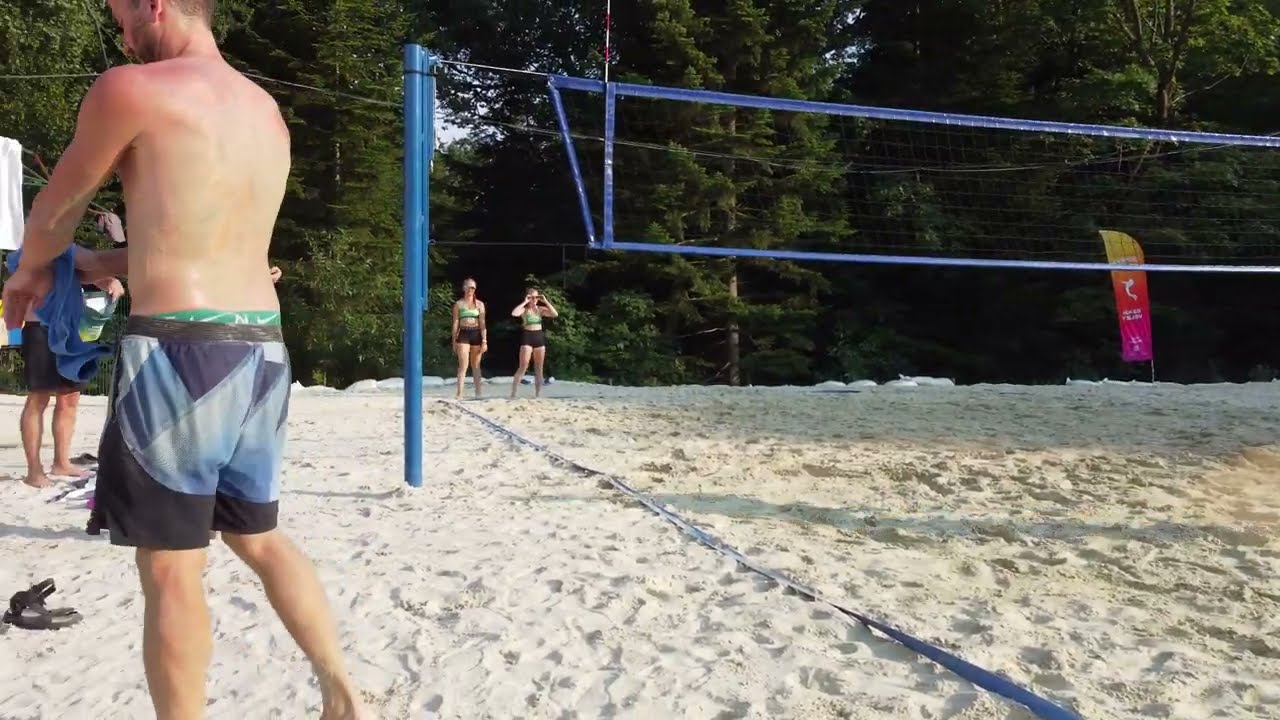In this photograph of an outdoor sand volleyball court, the ground is covered in white sand, and the court is divided by a blue net at the center. Two women are positioned at one end of the net, both dressed in matching outfits: black swim shorts paired with bright green swim tops. One woman sports sunglasses, while the other wears a visor. On the left side of the court stands a shirtless man, his back to the camera, wearing only blue and black swim trunks with green highlights and showing signs of sunburn on his shoulders. His environment is enhanced with a pair of sandals placed on the sand nearby. Adjacent to the court, a banner adorned with purple, red, and yellow colors advertises the sand volleyball event, and towering green trees provide a lush backdrop.